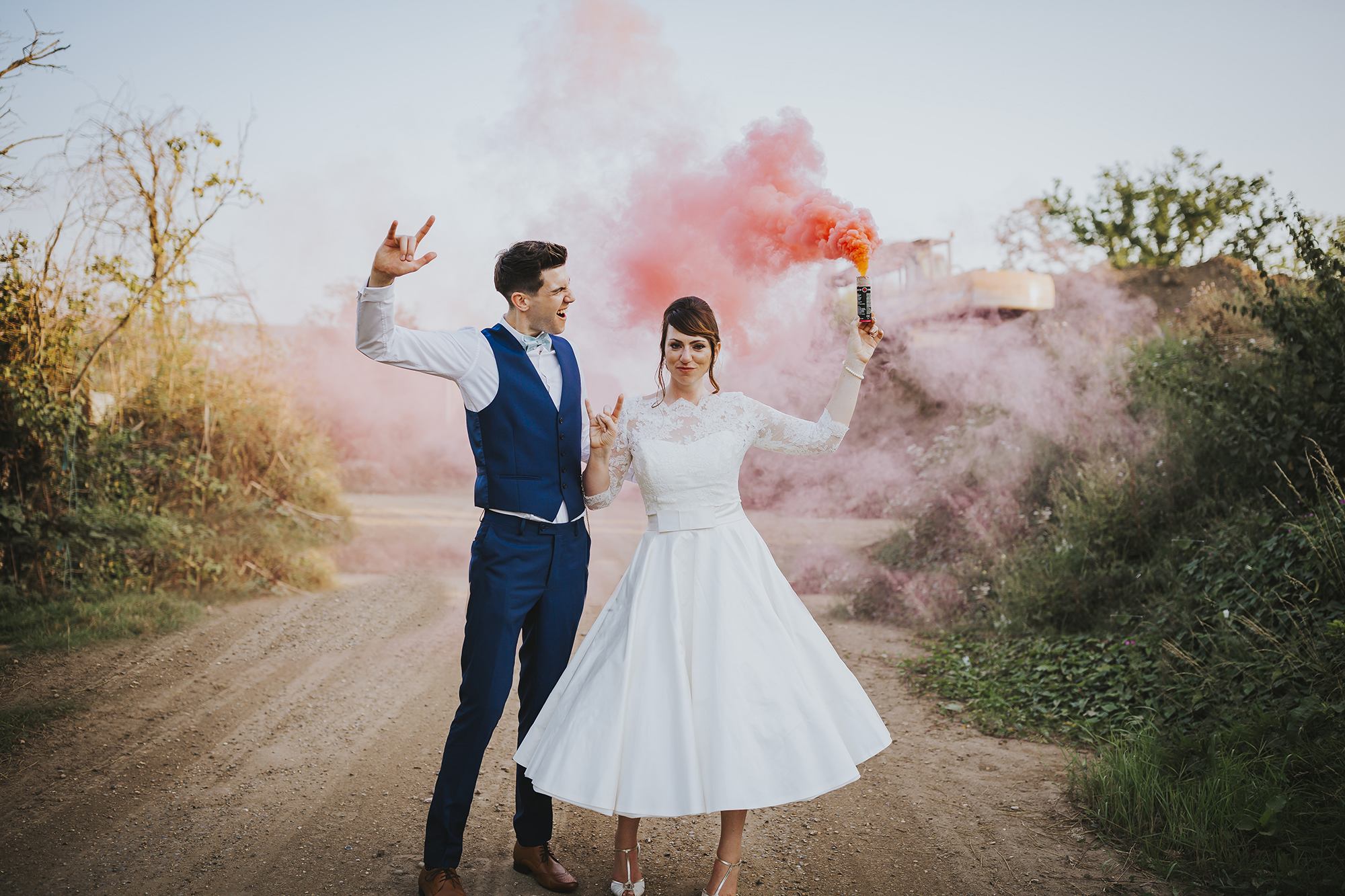In this vibrant image, a jubilant couple stands in the middle of a dirt road, surrounded by lush green vegetation on hillsides flanking either side. The woman, dressed in a stunning, full-length white gown reminiscent of a wedding dress, exudes confidence as she smiles directly at the camera. She is holding a flare stick in her left hand, emitting a striking orangey-red smoke that adds a vivid splash of color to the scene, her arm bent at a confident 90-degree angle. Simultaneously, her right hand is raised in a 'devil horns' gesture. Beside her, on her right, stands a man clad in blue pants and a matching blue vest over a white collared shirt, completing his attire with brown loafers. He mirrors her celebratory pose with his right hand also forming the 'devil horns' as he faces her, exclaiming his excitement. The sky above them is a muted blue-gray, providing a contrasting backdrop to their apparent festivity, possibly a gender reveal celebration. White high heels on the woman and the duo's expressive gestures capture a moment of shared joy and celebration.